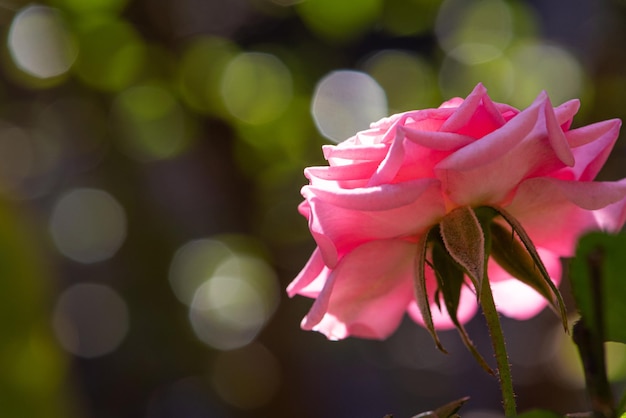This is a close-up landscape photograph featuring a single pink rose prominently positioned on the right-hand side of the image. The rose, with its large, pointed petals of a light to medium baby pink hue, is in full bloom and beginning to show signs of aging, with some petals curling underneath. Sunlight strikes the petals from the right, causing portions to appear almost whitish in spots due to the reflection. The stem, a dark green, supports the slightly drooping flower, contrasted by some brown and green leaves hanging down. The photograph's background is deliberately blurred, creating a bokeh effect with circles of green, gray, yellow, and black, which accentuates the rose as the focal point of the image.